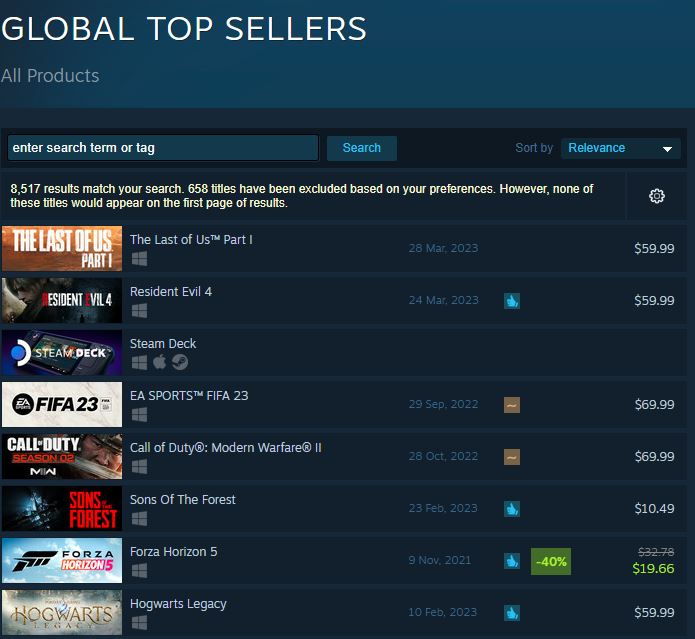Here is a cleaned-up and detailed caption for the image described:

---

This is a detailed screenshot of a website showcasing its global list of top-selling video games. The webpage is titled “Global Top Sellers - All Products,” and features a search bar labeled “Enter search term or tag,” allowing users to sort the listings by relevance. According to the site, there are 8,517 results matching the current search criteria, with 658 titles being excluded based on user preferences.

The image prominently lists the following top-selling video games, accompanied by their prices and additional details:

1. **The Last of Us Part 1** - $59.99
2. **Resident Evil 4** - $59.99
3. **Steam Deck** - Price not displayed
4. **FIFA 23** - $69.99
5. **Call of Duty: Modern Warfare 2** - $69.99
6. **Sons of the Forest** - $10.49
7. **Forza Horizon 5** - $19.66 (currently on sale with a 40% discount)
8. **Hogwarts Legacy** - $59.99

In the middle column, the screenshot shows dates presumably indicating either the release dates or the dates when these titles went on sale.